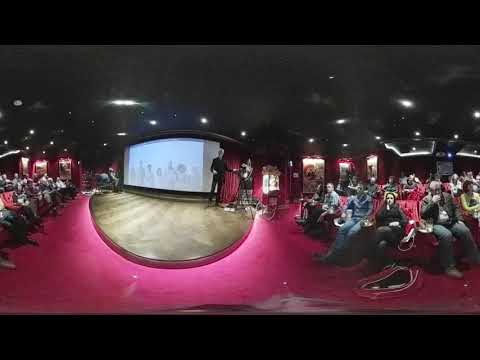The image appears to capture a presentation in a dimly lit, intimate theater setting with a black ceiling adorned with white pot lights. The focal point is a man dressed in an all-black suit standing on a slightly elevated, semi-circular brown stage, holding something in his right hand. The flooring of the room is carpeted in red, coherent with the red theater chairs arranged in rows for the audience. The scene behind the presenter includes a large curved screen that might be projecting a film or a solid image. Additionally, there are posters flanking the screen on both the left and right sides. The audience, which is well-lit, is seated and attentively facing the stage. The panoramic nature of the image creates a slight fisheye effect, blurring the background and making the stage appear more rounded. The overall ambiance suggests a possible work event or team-building exercise, captured in a cozy, theater-like environment.